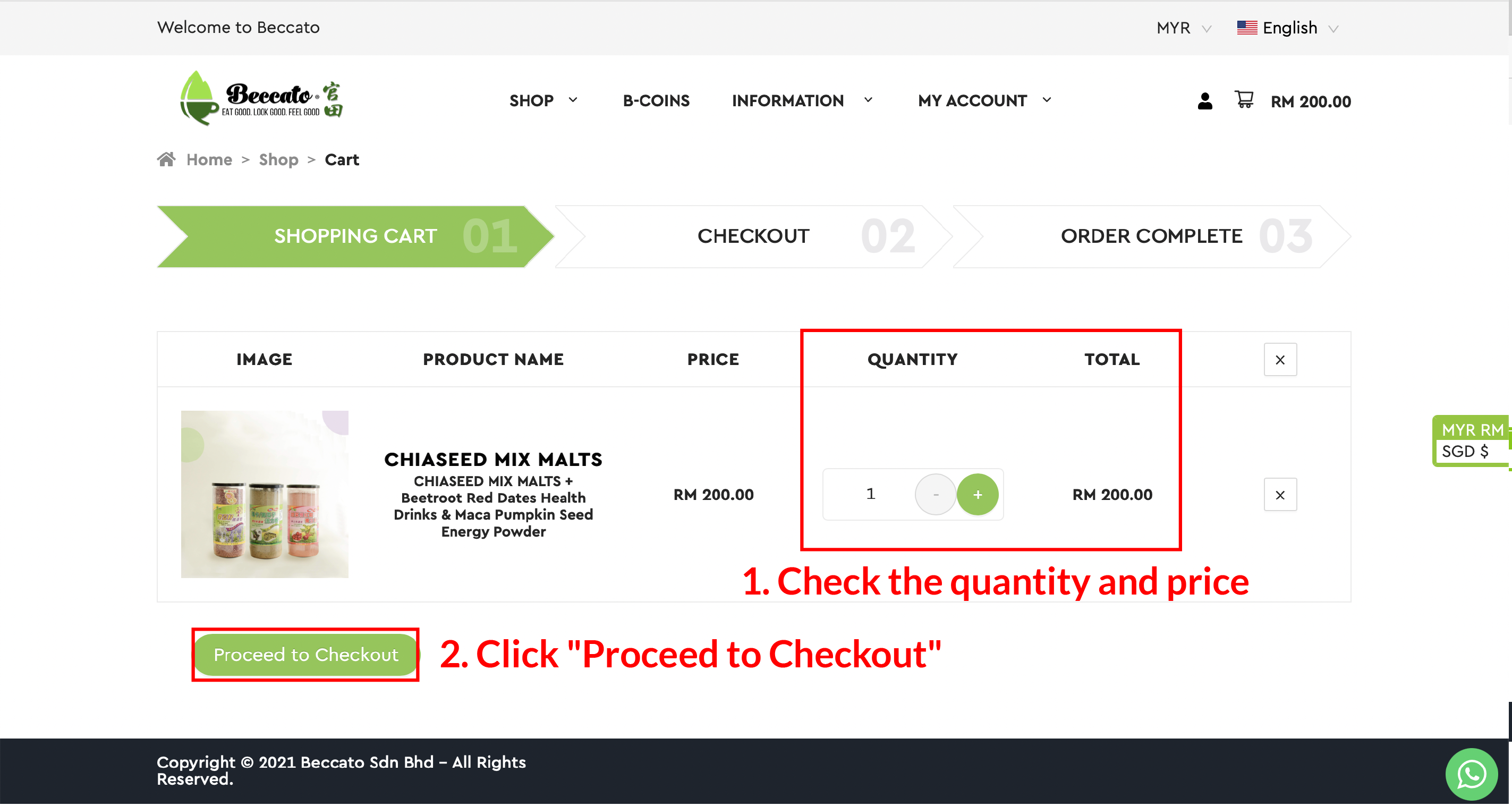The webpage features a prominent "Welcome to Bekato" message displayed at the top left corner alongside the Bekato logo. The company's slogan, "Look Good, Feel Good," is also prominently shown. At the top right of the page, there are several drop-down menus labeled "Shop," "Information," and "My Account," accompanied by smaller hyperlinks such as "Bitcoins" and language selection options. The language is set to English, indicated by an adjacent USA flag icon.

The navigation directory indicates the current path: "Home > Shop > Cart." Below this breadcrumb trail, various cart elements are displayed, including columns titled "Image," "Product Name," "Price," "Quantity," and "Total." At the bottom of the page, a footer notes the copyright: "© 2021 Bekato SDN PhD. All rights reserved."

The detailed organization of the webpage provides a comprehensive view of Bekato’s online shopping interface, highlighting its user-friendly navigation and international adaptability.